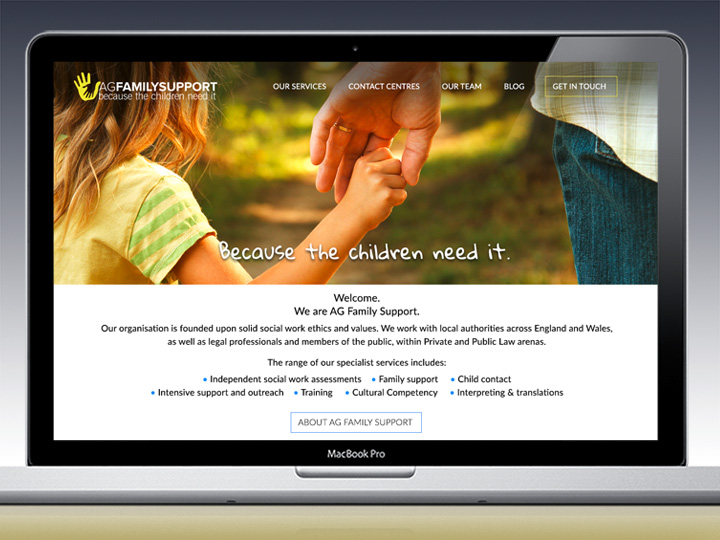The image depicts a MacBook Pro with a dark gray background, displaying the website of "AG Family Support." The website features a prominent banner, which shows a touching scene of a child reaching up to hold an adult's hand. The child's face is not visible, revealing only her hair and a part of the adult's hip, highlighting a sense of support and care. 

The navigation menu of the website includes tabs labeled "Our Services," "Contact Centres" (spelled in British English), "Our Team," "Blog," and "Get in Touch." Below the banner, the screen is divided into two halves. The bottom half features a white square with the text "Because the children need it" followed by a welcoming message: "Welcome. We are AG Family Support." This section further elaborates on the organization's focus areas and the services they offer, concluding with a section titled "About AG Family Support."

In the background of the MacBook Pro screen image, the tip of the laptop's keyboard is barely visible, adding to the overall composition.